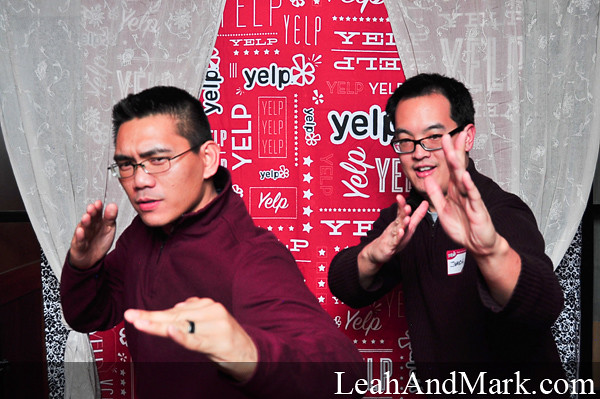In this photograph, two Asian-American men in their 20s or 30s are prominently featured against a backdrop heavily branded with the Yelp logo in various fonts and colors. Both men are wearing glasses and have short black hair. They are positioned with their hands raised as if poised in a karate stance, adding an element of playful energy to the image.

The man on the left sports a maroon zip-up sweatshirt and has a subtle smile, while the man on the right wears a black long-sleeved shirt adorned with an unreadable name tag. They both look directly at the camera, seemingly engaged with the viewer. The background, primarily gray with a prominent red central section displaying the Yelp logos, is flanked by sheer, possibly lace, curtains. This setting suggests it might be part of a photo booth, potentially at an event or promotional activity, given the presence of the website LeahandMark.com in the bottom right corner.